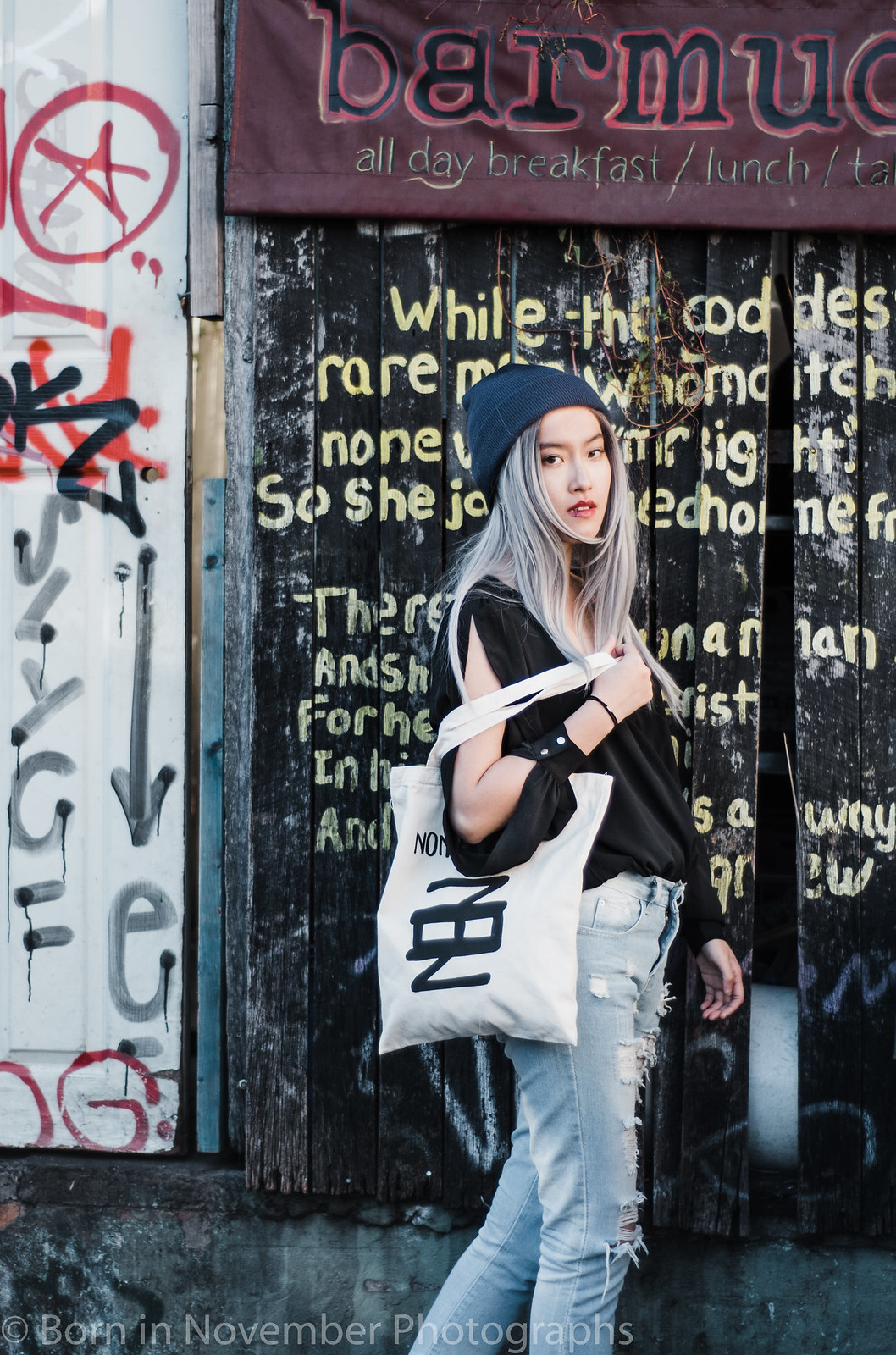In this vibrant street photo, a stylish model is captured in mid-stride, walking from left to right. She is an Asian woman with striking, dyed gray hair, tucked under a blue winter beanie that complements her trendy look. Her makeup includes noticeable red lipstick, enhancing her delicate features. She’s dressed in a black long-sleeve blouse with open slit sleeves, effectively showcasing her right arm, which bears a white tote bag. The tote bag features distinctive black lettering and a rectangular design, although its full details are obscured. She pairs her top with ripped light blue jeans, tattered at the thigh, adding to her edgy fashion sense.

The setting appears to be the exterior of a restaurant named "Bar Moody," discernible from a partially visible maroon sign above, proclaiming "All Day Breakfast and Lunch." The woman stands in front of black slats covered in yellow graffiti, which she partially obscures, though a peace sign inside a circle is visible at the top left of the image. The ground beneath her appears to be concrete, with faint white text reading "Born in November Photographs." Behind her, graffiti-laden walls contribute to the vibrant, urban atmosphere of the scene.